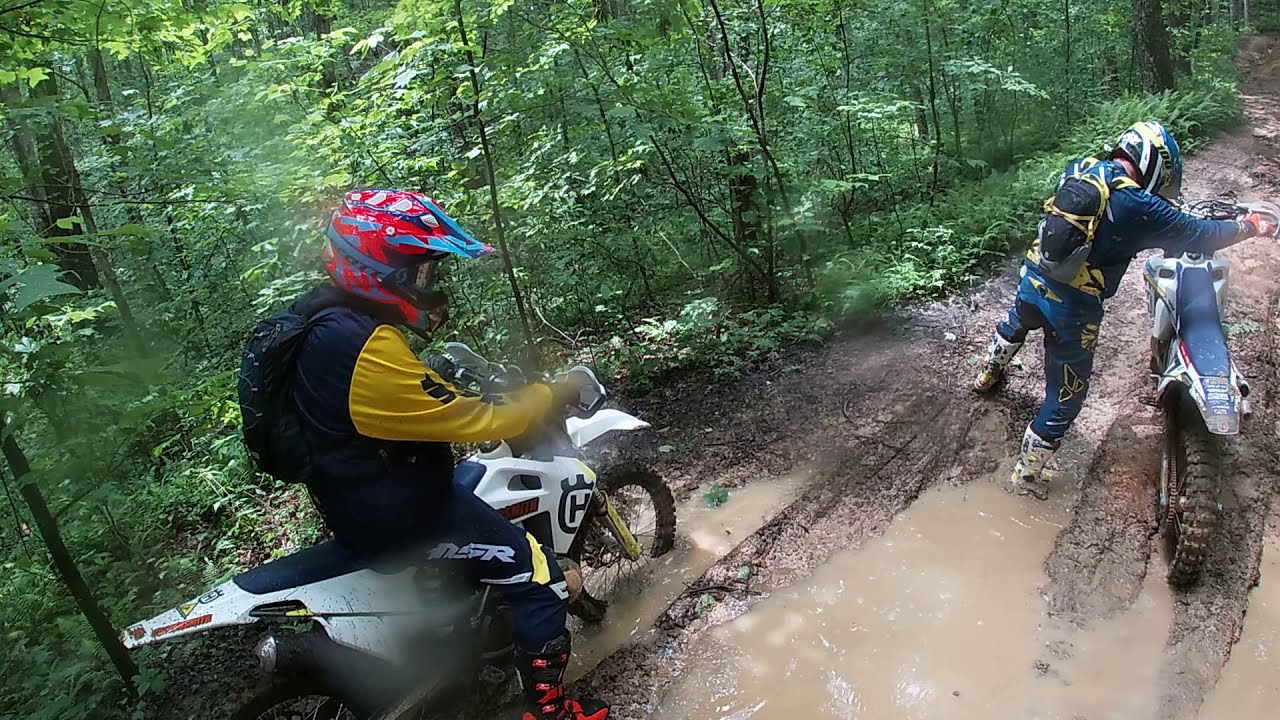In this horizontally aligned rectangular photograph, two dirt bikers navigate a muddy forest trail surrounded by trees with bright green leaves and dense underbrush. The biker in the foreground, seen slightly to the left, is wearing a distinctive red helmet with a blue bill, a navy blue top with yellow long sleeves, and is seated on a predominantly white motorcycle with black and red accents. This rider has stopped, with their feet on the ground, immersed in the muddy, brown puddles, preparing to push their bike through the standing water. The second biker, positioned more to the right, donning blue and yellow gear with a matching backpack and a white and blue helmet, is off their blue and white motorcycle, actively pulling the bike out of one of the deeper puddles. The elevated perspective of the image captures the rugged, rustic nature of the trail and the challenges posed by the thick mud and water for these determined riders.